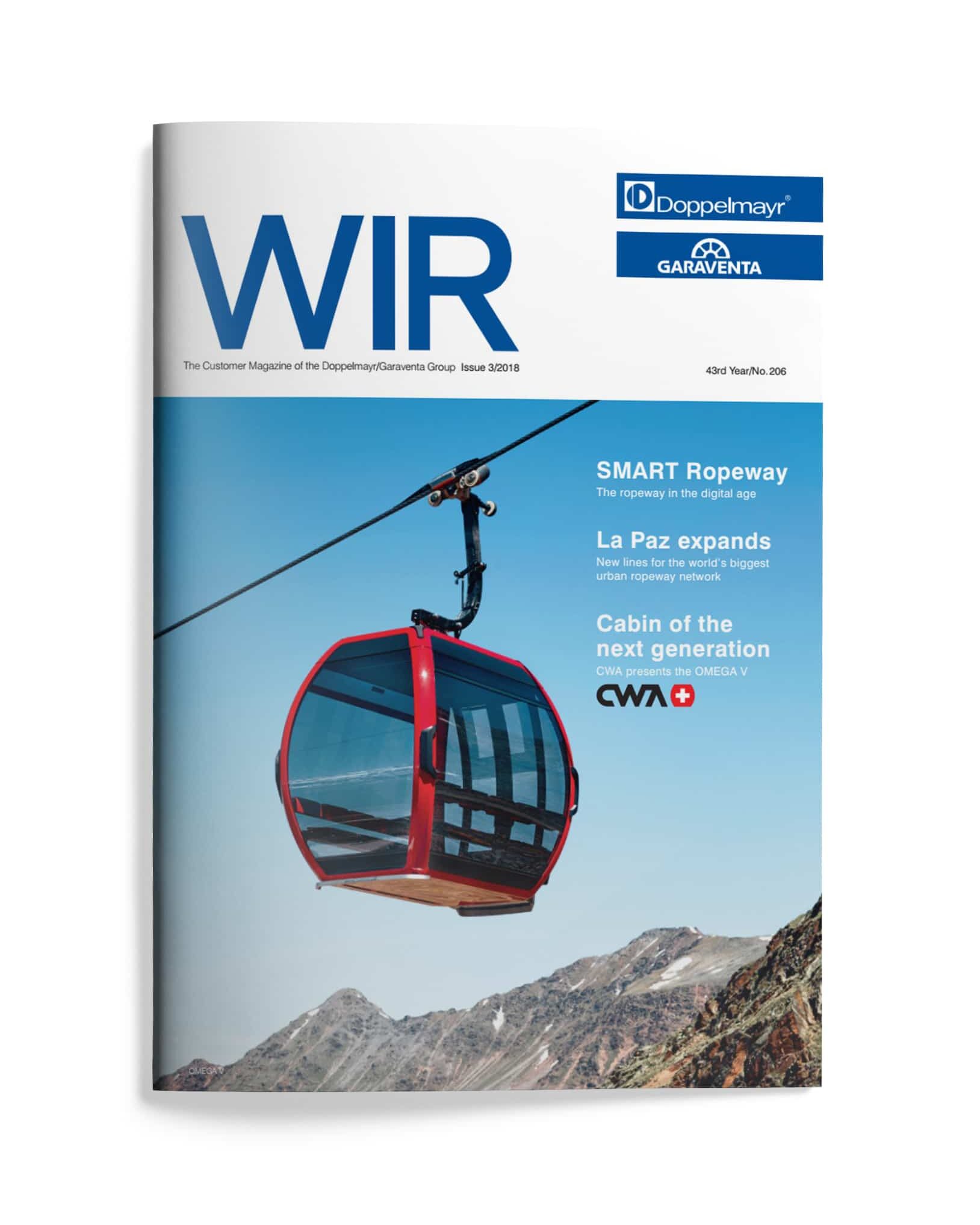This is a vertical-rectangular magazine cover. The top section has a white background with the magazine's title, "WIR," prominently displayed in large blue letters. Below the title, small black text reads, "the customer magazine of the Doppelmayr Garaventa Group," followed by "Issue 3/2018." In the upper right corner, there are two blue rectangles with white text; one reads "Doppelmayr" with a small logo to its left, and the other reads "Garaventa" with a logo above it.

The majority of the cover features a photograph of a modern, enclosed cable car with a red metal frame and glass walls, moving over a mountainous landscape. The mountains below are primarily composed of gray stone with patches of lingering snow. On the right side of the image are several white text captions announcing the magazine's articles: "Smart Ropeway," "La Paz Expands," and "Cabin of the Next Generation."